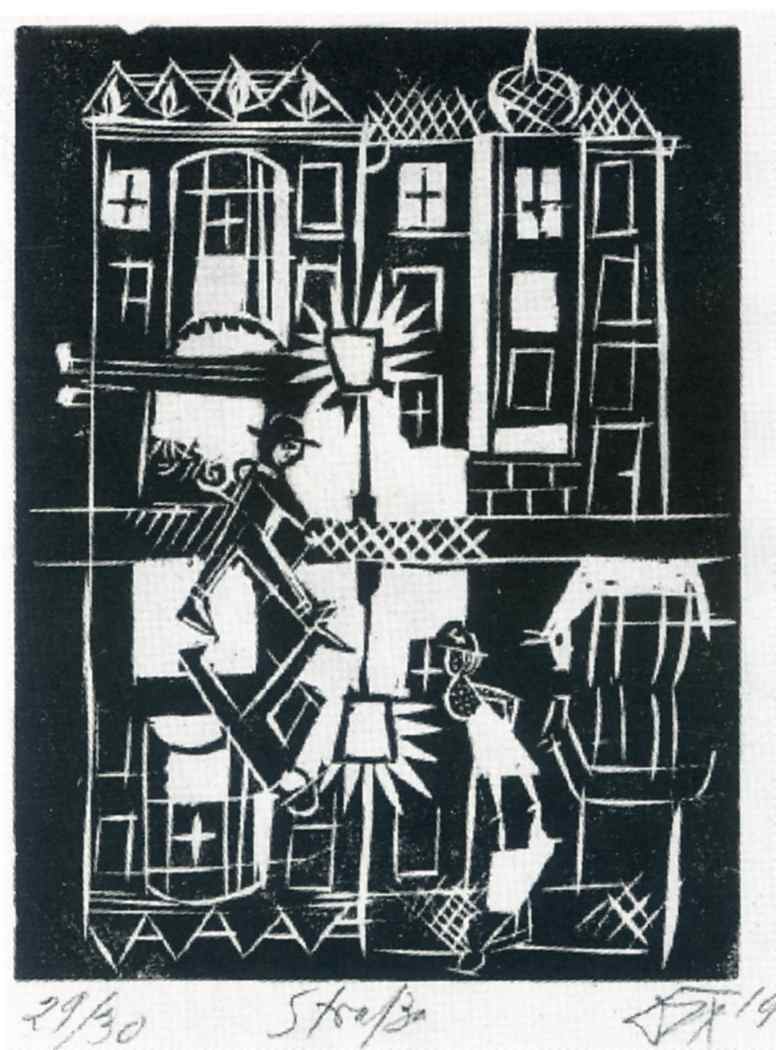This detailed black-and-white print, titled "29 out of 30" and attributed to an artist named Straitza in 2019, depicts a vertically aligned, rectangular scene dominated by a tall, six-story house. The background is predominantly black with intricate white highlights. On the top floor of the house, the windows feature small black crosses within white panes, suggesting a pattern of light and shadow. At the bottom of the print stands a girl, distinguished by her triangular, white dress and a smiling face beneath what appears to be a hat. To her right, a mother-like figure dressed entirely in black, also wearing a hat, seems to be pushing something as she leans forward. Centered in the scene is a lamppost radiating white rays of light, creating a focal point that illuminates both the upper and lower sections. A father figure, depicted in front of the lamppost, steps forward with an intense expression. Completing this dense composition is an animal, possibly a horse with horns, grazing near the girl on the right side. The overall artwork carries a surreal and somewhat chaotic feel, making it a captivating piece in any personal portfolio.